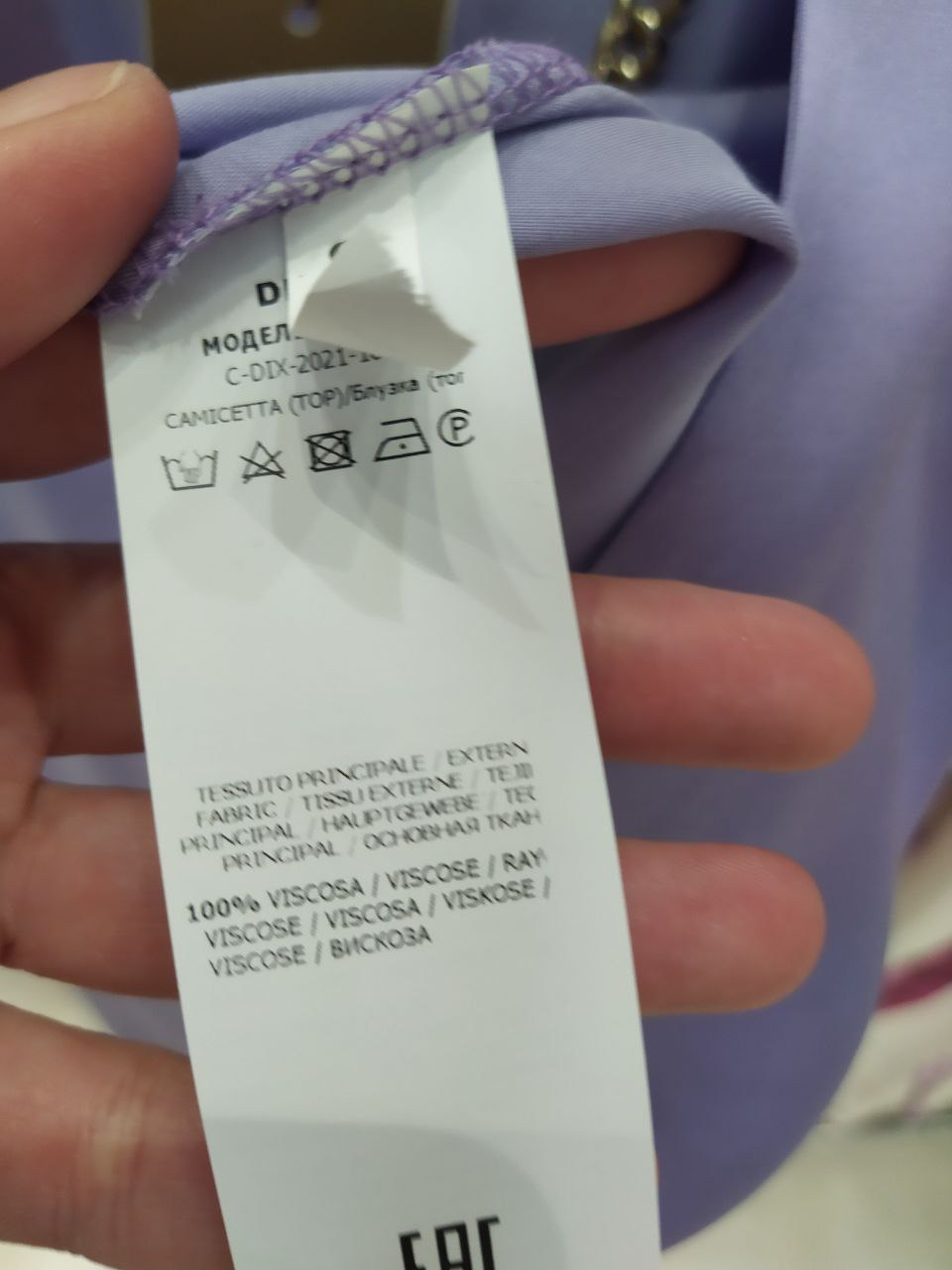A close-up image captures a lavender-colored garment, with a focus on the clothing tag. The tag, predominantly written in Russian, also features snippets of text in multiple languages including English, where words such as "fabric" and "ray" can be deciphered. The specific type of garment is unclear due to the tight framing, but the soft texture and color suggest it might be a blanket, sweater, or some other kind of top. A hand gently holds a portion of the fabric, slightly lifting the tag to make its details more visible. The lighting highlights the subtle hues of the lavender textile, adding a calm and cozy atmosphere to the scene.